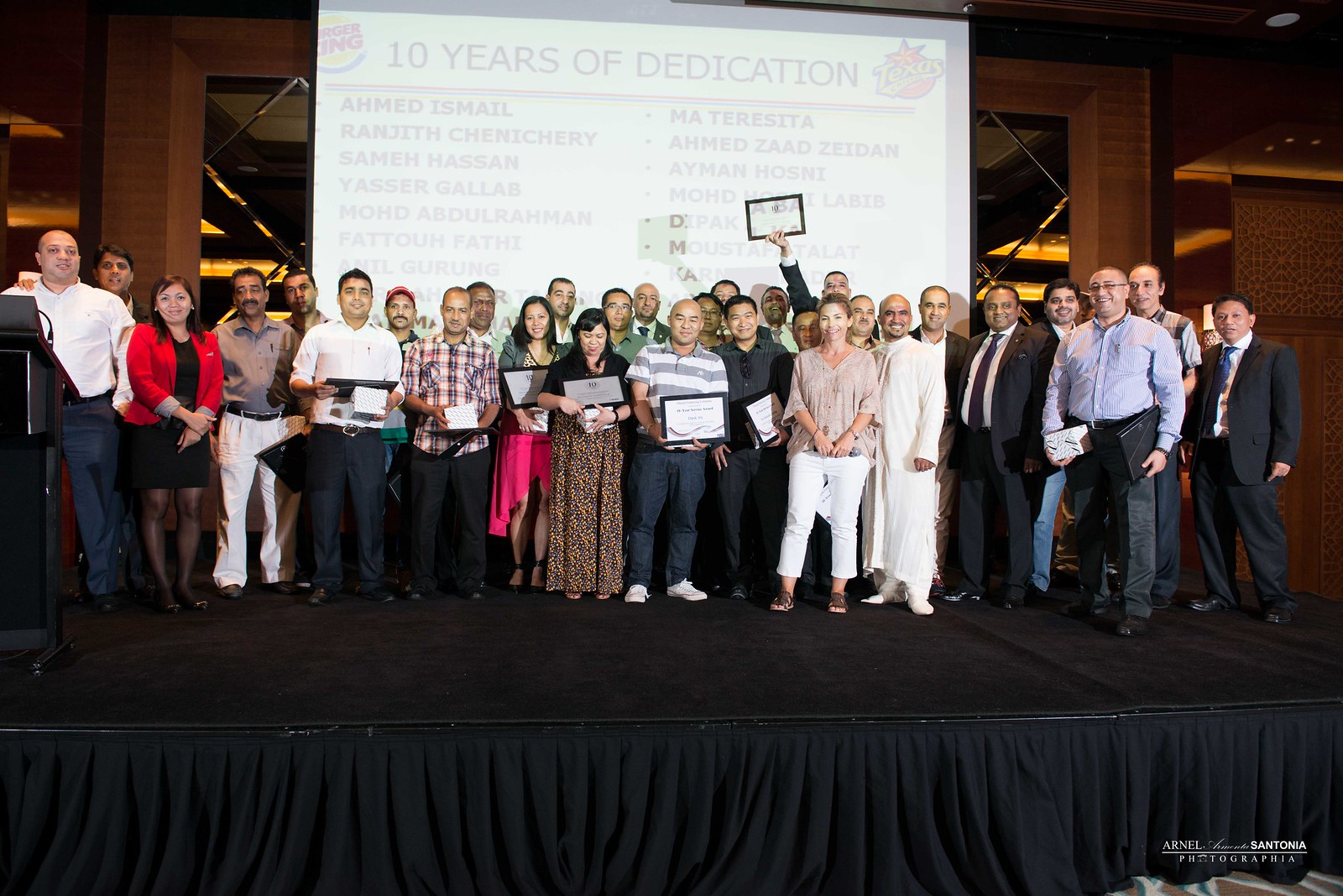A large group of about 20 to 25 men and women are standing on a black stage, posing for a celebratory photo. Center-stage, a few individuals proudly hold up certificates or plaques, reminiscent of a graduation ceremony. The participants are a mixture of various ethnic backgrounds, predominantly Middle Eastern, South Asian, and possibly East Asian. They are attired in a range of outfits from suits and ties to button-down shirts and polo shirts, with one man notably dressed in a white robe and slippers. 

The backdrop features a large projector screen displaying a message that reads "10 Years of Dedication," flanked by the Burger King logo in the top left and the word "Texas" in the top right. Below this message is a list of names such as Ahmed Ismail, Ranjit Chennacheri, Sameh Hassan, Yasir Ghalab, Maa Teresita, and Ahmed Zahed Seydan, hinting at a diverse group of honorees. The atmosphere is one of joy and pride as the group stands in a well-lit large ballroom, complete with a podium on the left side, ready to celebrate their collective achievements.